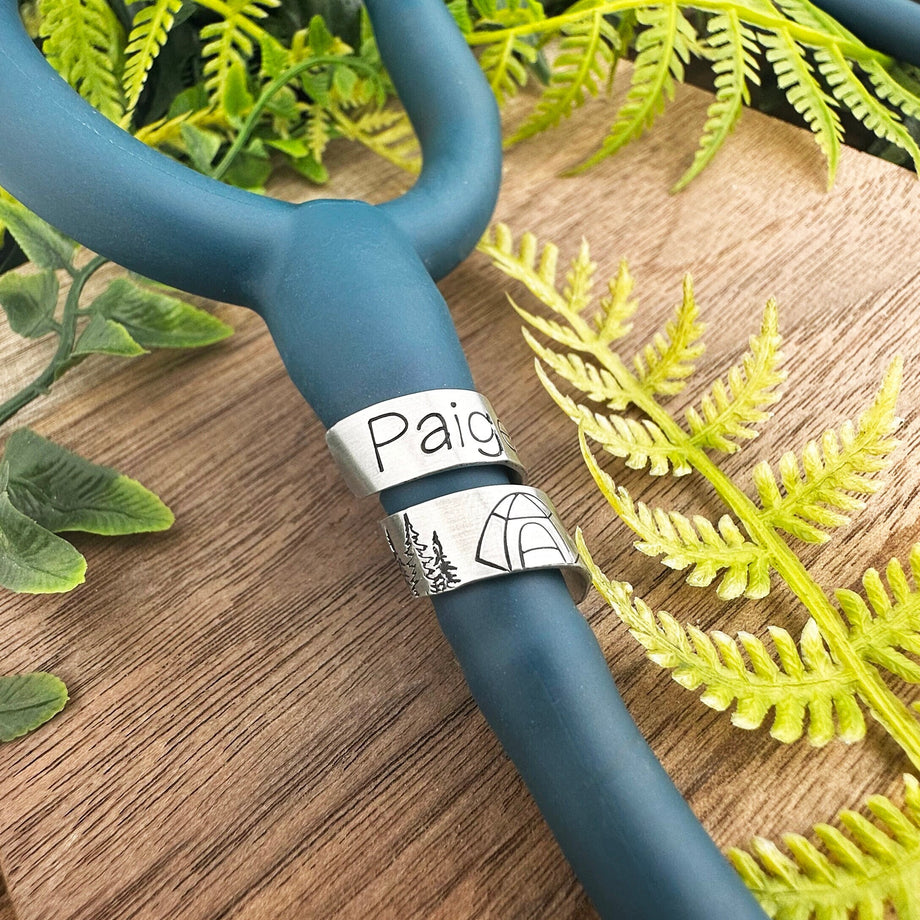This is a detailed color photograph of an outdoor camping tool, likely a tent peg or shovel handle, positioned atop a wooden grain tabletop. The dark blue-green cylindrical body of the tool, made of either molded rubber or plastic, lies horizontally in the image. Attached to the handle are two white tags: the upper tag reads "PAGE" in black lettering, while the lower tag features black images of three pine trees and a camping tent.

Surrounding the central object are various plants, including a few yellowing ferns that suggest they are past their prime. There are also other types of foliage, with some lighter green leaves likely from the same plant and a darker green vine-like plant on the left. The photo clearly shows the intricate grain patterns of the stained wooden surface beneath the tool, enhancing the natural aesthetic of the scene.